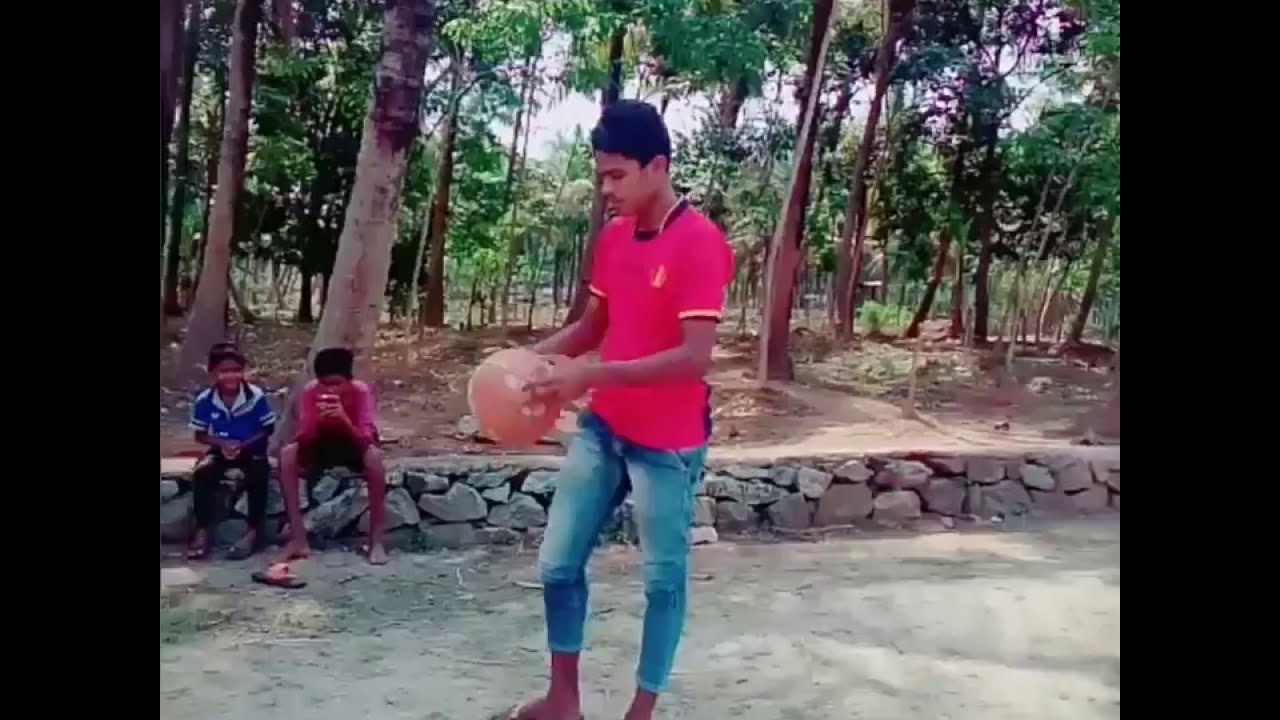This slightly blurred horizontal photograph, bordered by thick vertical black edges, captures a daytime outdoor scene with earthy textures. At the center stands a man with short black hair and brown skin. He wears a red short-sleeved polo shirt featuring gold and blue collar fringes, and blue jeans that are rolled up at the bottoms. He's holding a brown, somewhat indistinct ball, and his feet are mostly cut off from the image, although a hint of sandals or flip-flops can be seen. The man is positioned on a light gray, rocky dirt ground.

On the left middle of the image, two younger boys sit on a low stone wall made of gray stones. One boy, who has slightly darker skin and short black hair, wears a blue polo shirt with white stripe details on the sleeves and black pants. The other boy, dressed in a red shirt and black shorts, is more blurred but similarly has slightly darker skin and short black hair. Neither boy's shoes are visible.

In the background, stretching from left to right, is a dense cluster of tall tree trunks with green leaves, and patches of the light sky can be seen filtering through the foliage. The ground throughout the scene is predominantly dirt and rocks, adding to the rustic outdoor atmosphere.